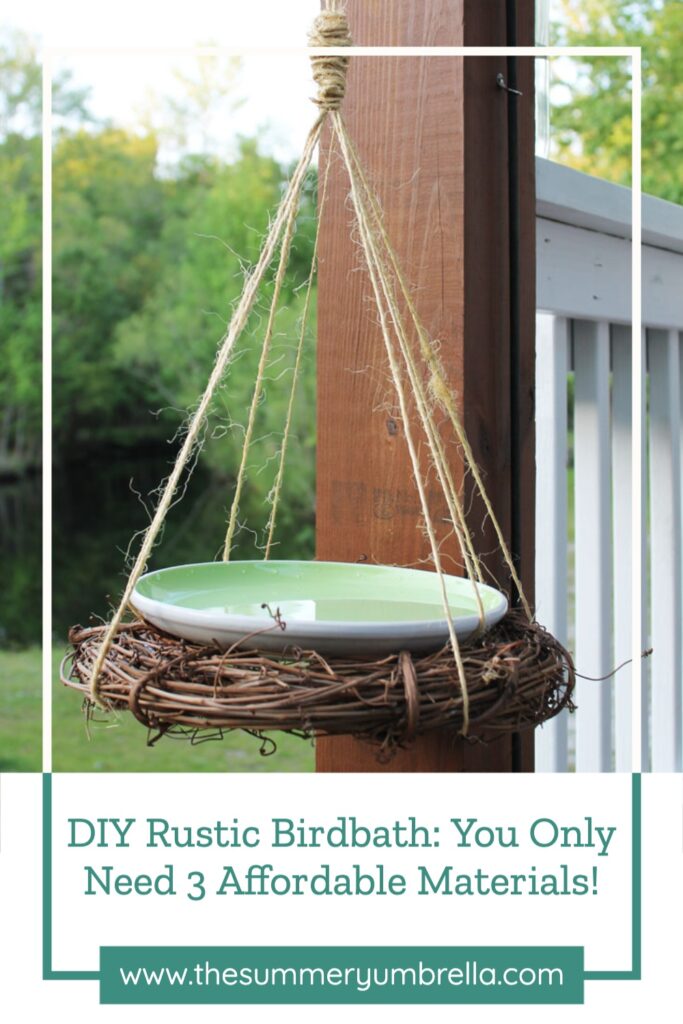The image is a color photograph in portrait orientation, featuring a DIY rustic birdbath hanging from a porch. The birdbath is suspended by a knotted twine rope that splits into seven strands, fanning out in a pyramid shape to support a flat, woven twig platform. On this platform rests a light green saucer filled with water. Behind the birdbath is a dark wooden post attached to a white handrail, with vertical white pickets below. A grassy backyard with dark green trees can be seen to the left, and more trees are present in the top right corner. The bottom of the image includes a white rectangle with teal text stating "DIY Rustic Birdbath: You only need three affordable materials!" Below that, in a green rectangle with white text, is the website "www.thesummeryumbrella.com." The overall style blends photographic realism with graphic design elements.